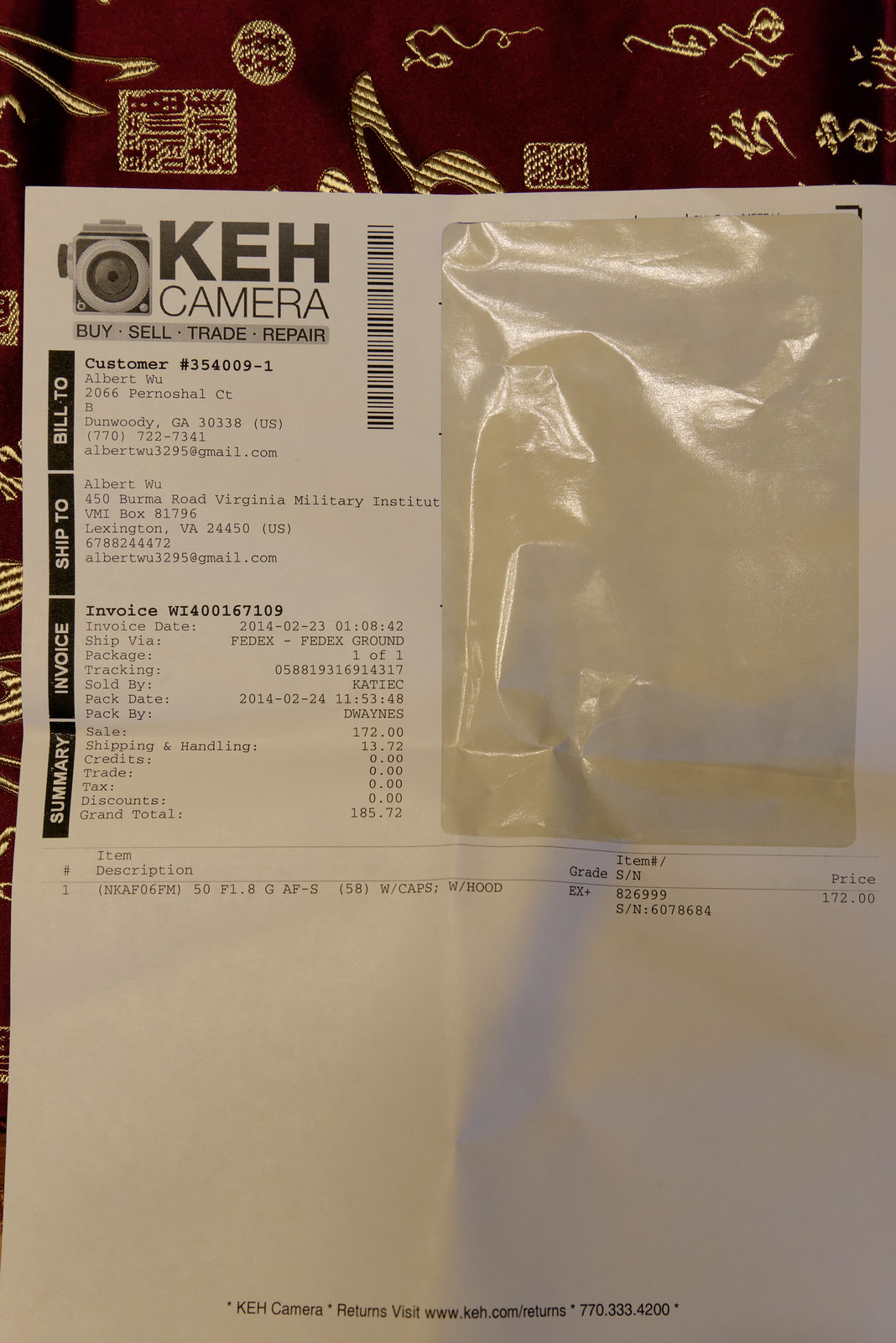The photograph is of a paper receipt with significant details indicating it's an invoice from KEH Camera. The top right corner of the receipt shows evidence of a sticker that has been removed, likely containing shipping or address information. The left side of the receipt prominently features the KEH Camera logo, accompanied by the tagline "buy, sell, trade, repair." Below this, the receipt lists a customer number, "354009-1," and the cusomter's name, Albert Wu. The stated billing address is "20066 Financial Circle, Dunwoody, Georgia," while the shipping address is "Lexington, Virginia." Both addresses are for Albert Wu, indicating a different billing and shipping address for the same person. 

Further down the left side, the receipt includes sections labeled "bill to," "ship to," "invoice," and "summary." The cost summary indicates a grand total of $185.72, with the item purchased being a camera with caps and hood, priced at $172.00 before shipping costs and showing no tax. The item was shipped via FedEx Ground. Additionally, the bottom of the receipt mentions a kit camera, providing a thorough breakdown of both the financial and logistical details concerning the shipment.